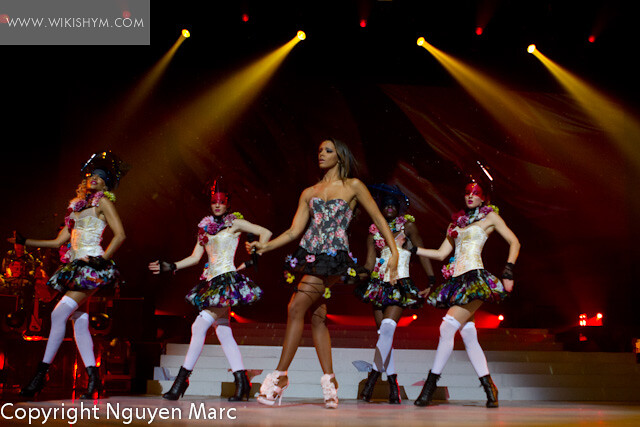This photograph captures the dynamic energy of a live performance. At the center, a female singer in a strapless floral dress and pink high heels dances towards the left of the stage. Surrounding her are four backup dancers, all perfectly synchronized. The dancers are adorned with intricate headpieces—two in red and two in blue—each partially covering their faces and adding an avant-garde element to their appearance. They wear white bustiers, floral skirts, white thigh-high stockings, and black high heels. The stage itself is dramatic, featuring black and red steps that rise behind the performers. Overhead, large yellow stage lights beam down, creating a vibrant atmosphere. In the top left corner of the image, the URL "www.wikishim.com" is displayed in a translucent gray box. This detailed snapshot captures both the individual flair of each performer and the cohesive visual spectacle of the performance.